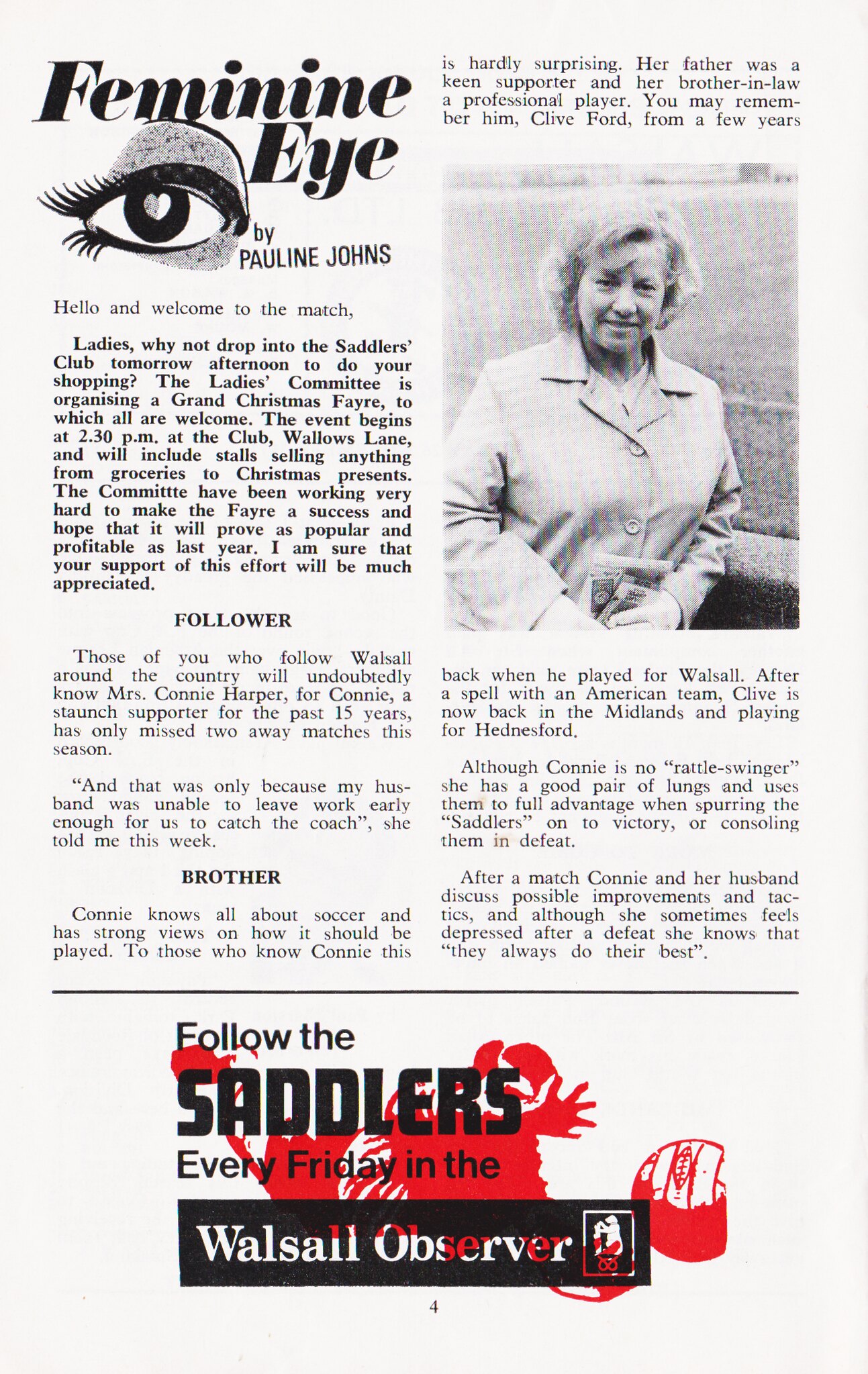This page appears to be from a magazine, primarily in black and white. At the top left, the title "Feminine Eye" is written in bold black text, attributed to Pauline Johns. Underneath the title, there is a close-up artistic drawing of an eye with elongated eyelashes and a heart-shaped pupil. Below this illustration, the article begins with the attention-grabbing phrase, "Hello and welcome to the match."

The article features two columns of text. The left column includes sections labeled "follower" and "brother" and begins with a welcome message encouraging ladies to drop by the Sadler's Club for a grand Christmas fair organized by the ladies' committee. The right column starts with a brief paragraph followed by a black and white photograph of an older, middle-aged woman, who could be the author, Pauline Johns. She appears to have light hair, smiles faintly, and leans on an object while wearing a jacket, though the exact details are ambiguous due to the black and white format.

At the bottom of the page, there is a colored section that prominently reads "FOLLOW THE SADLER'S" in large, rounded, black, stylistic capital letters. Below this, in regular text, it says "Every Friday." This is followed by a small black box with the phrase "Walsall Observer" in white letters, indicating the magazine's name. Behind this text block is a simple red illustration that is not clear enough to identify.